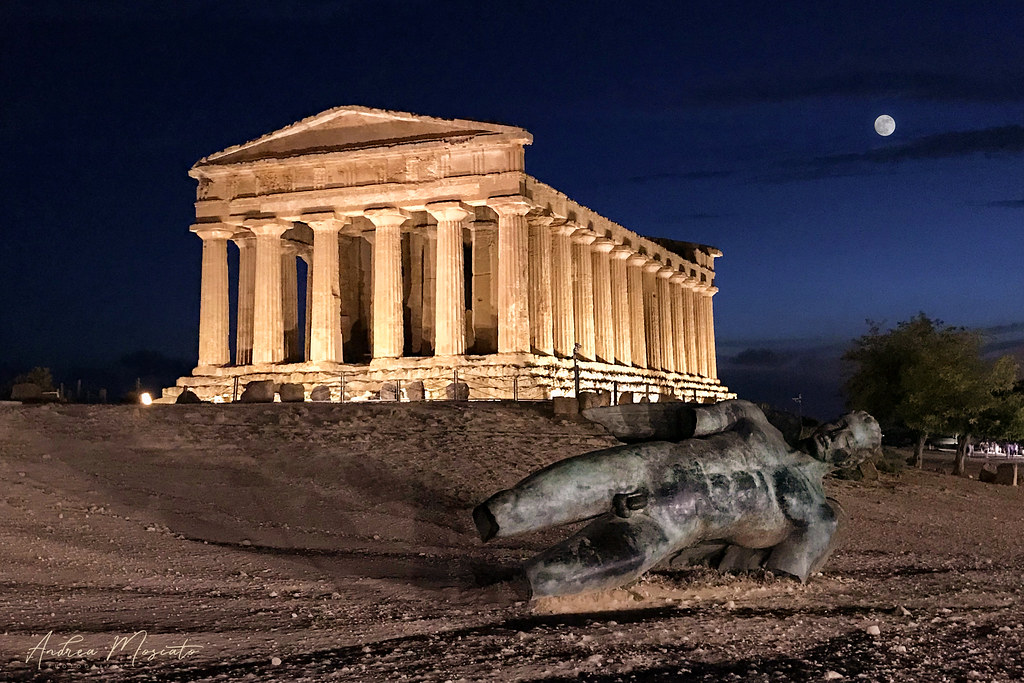This color photograph, captured by Andrea Moscato, portrays a captivating nighttime vista of a grand Roman architectural structure, possibly a temple or the Colosseum, illuminated against a dark sky with patches of blue and a full moon visible in the top right corner. The ancient structure, composed of white stone and numerous pillars, stands solemnly atop a brown, rocky dirt hill surrounded by a fence on the left side and trees on the right. In the foreground lies a broken statue of an anatomically correct, nude male figure, missing its arms from the elbows down and legs from the knees down, staring toward the viewer with closed eyes, further emphasizing the eerie, historical ambiance of the scene.